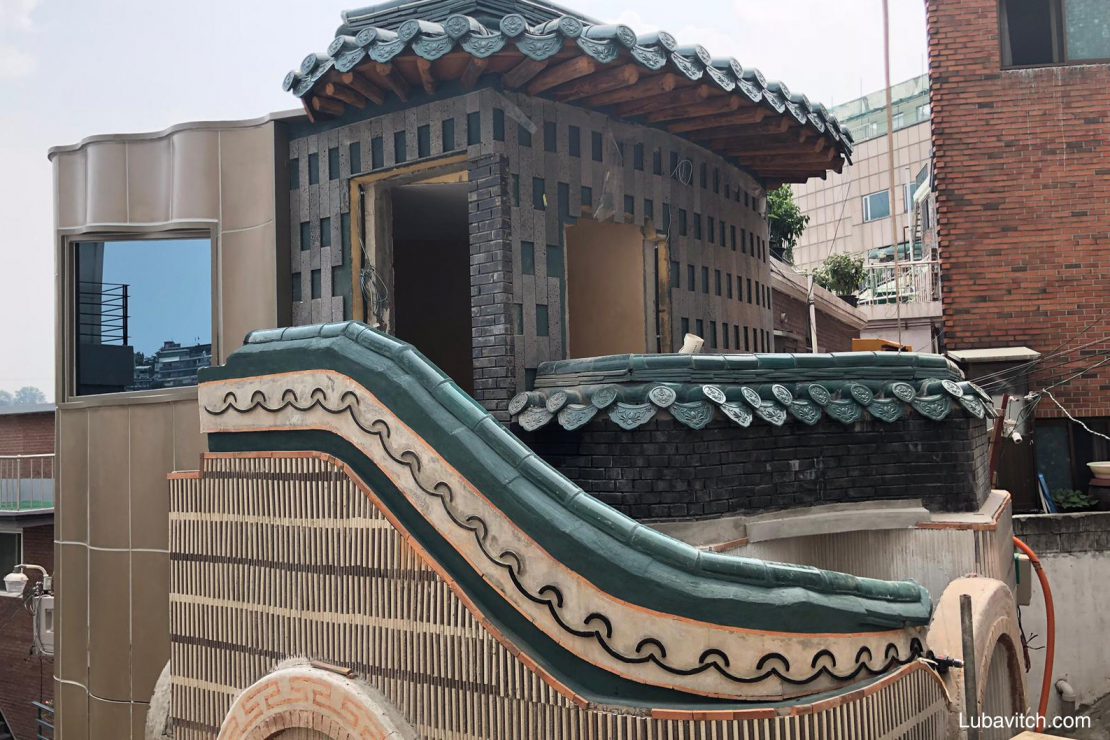The photograph captures a strikingly stylish and colorful futuristic building bathed in daytime light. The roof features an eye-catching circular or semicircular design, supported by logs and adorned with a draped blue edging around its outer circumference. Beneath the roof lies a square section of the building, distinguishable by its blue and white—or possibly blue and gray—facade, suggesting the use of stone. Prominently, there's a balcony at the forefront, decorated with the same draped blue edging and constructed from greenish-blue material, which could be stone or logs. An ornate teal staircase with a swirling pattern on its railing leads up to this balcony, continuing to a door of the building.

Adjacent to this main structure, a curvy building section featuring a large window and undulating beige surface hints at being part of the same architectural masterpiece. In contrast, to the right of this extraordinary building, a more conventional red brick building punctuates the scene, highlighting the unique and unusual design of the main structure. The entire scene exudes an unparalleled architectural charm, rendering it unlike anything typically seen before, set against the backdrop of a clear daytime sky.